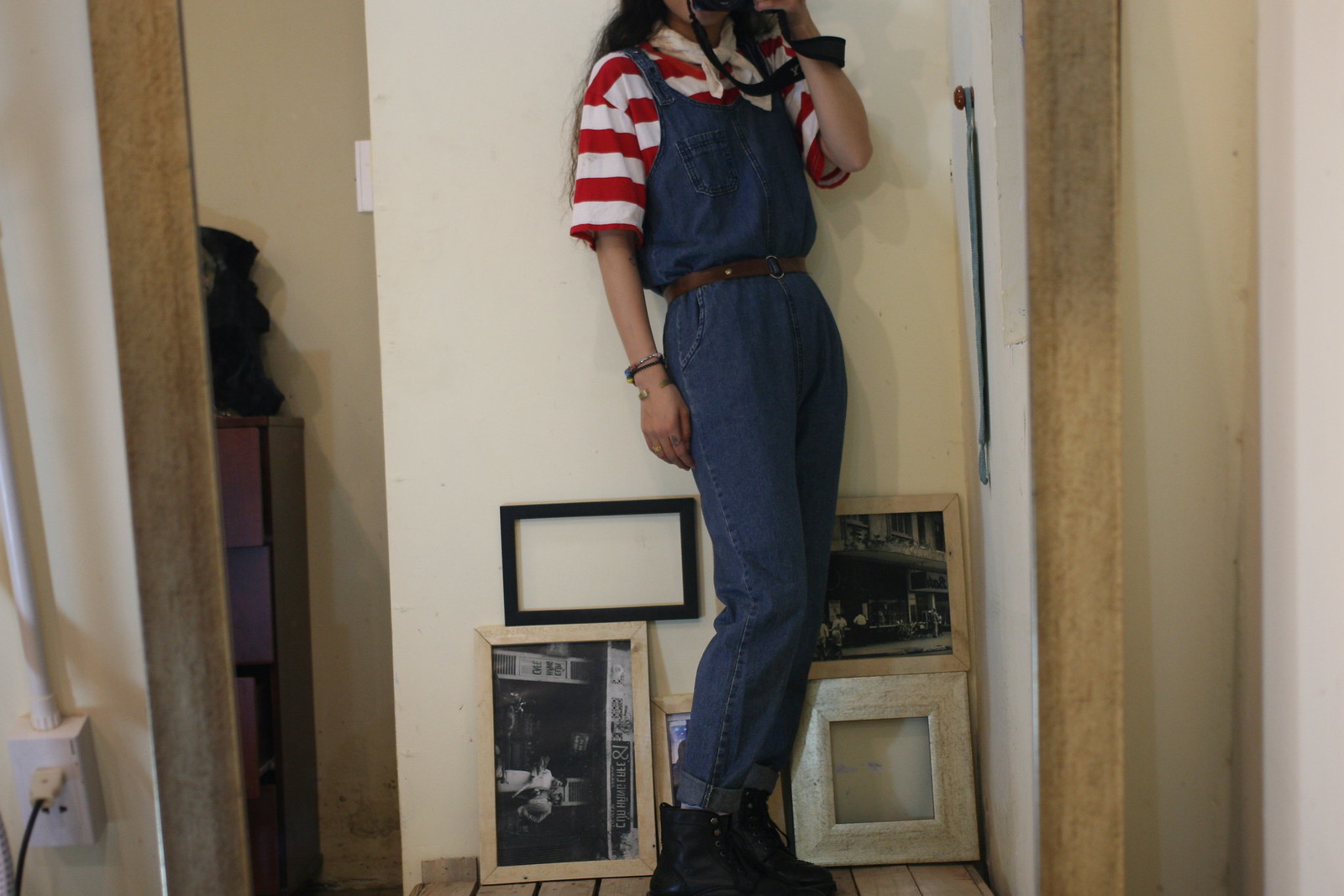The image captures a young woman with dark hair standing on a wooden crate, wearing blue denim overalls cinched with a brown leather belt, a red and white horizontally striped short-sleeve t-shirt with a white collar, and black leather combat boots. From her chin down, she is seen from a slightly angled perspective, emphasizing her right side and front. She accessorizes with a silver bracelet on her right wrist and has black sunglasses hanging from her arm. The background shows a white wall adorned with a variety of picture frames: a black rectangular frame, a beige rectangular frame with a black-and-white photo, another plain beige wooden frame, and a square white frame. To the far left, there is a doorway, a white pipe with an electrical outlet and a black cord plugged into it, and possibly a black dresser with purplish drawers. The ambient setting suggests an indoor space with a blend of unorganized decor and casual attire.